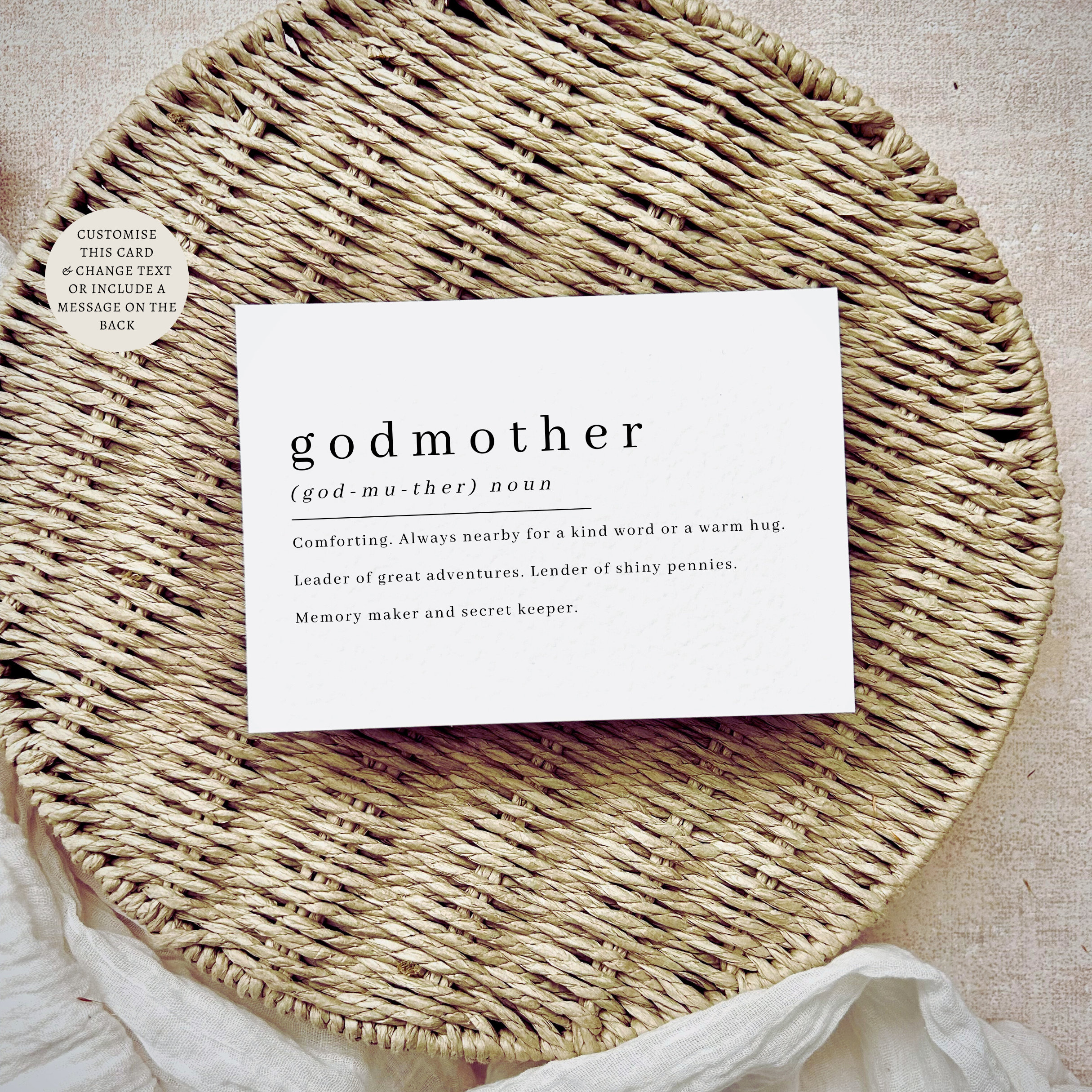In the photograph, a modern visual advertisement, the focal point is a round wicker basket with a white tan finish. At the center of the basket's lid, a white card prominently displays the word "godmother" in lowercase letters, followed by its phonetic pronunciation and definition. The definition reads: "Comforting, always nearby for a kind word or a warm hug. Leader of great adventures, lender of shiny pennies, memory maker, and secret keeper." The background is beige with a subtle cloth surface beneath the basket. In the upper left corner of the image, there is a circle containing the text: "Customize this card and change text or include a message on the back." This advertisement effectively showcases the custom card offering, likely intended for a small business or online shop.